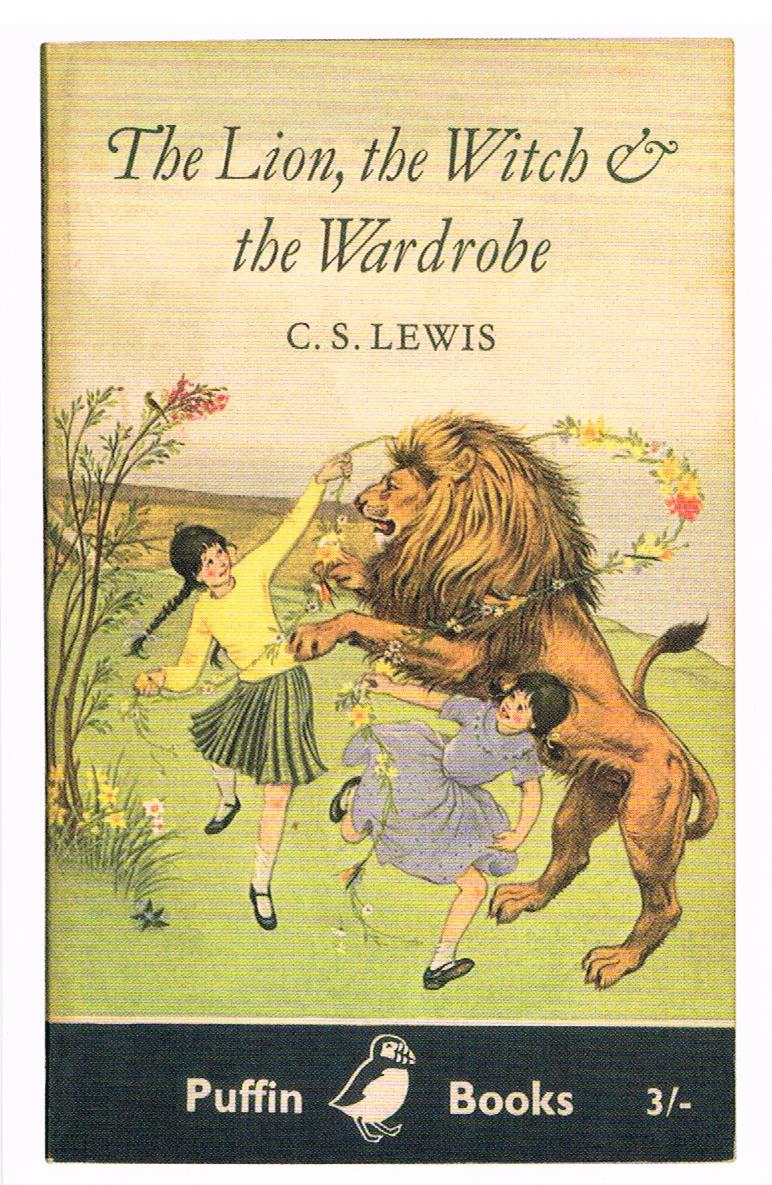The book cover for C.S. Lewis's "The Lion, The Witch, and The Wardrobe" features a nostalgic, old-fashioned design with a semi-cursive title at the top and the author’s name, C.S. Lewis, in all caps below it. The cover showcases an idyllic outdoor scene with lush green grass and a small tree with a blooming red flower on the left. Central to the imagery are two young girls and a majestic golden brown lion. The girl on the left, dressed in a long-sleeved yellow sweater and a green pleated skirt, holds one end of a flowering vine with her left arm raised. She has long, dark hair and black penny loafers. The girl on the right is dressed in a flowing light blue dress, also with dark hair and black penny loafers, and is looking over her shoulder at the girl in the yellow sweater. They are playing with the lion, whose grand mane and tail are elegantly displayed as he stands on his hind legs, appearing to dance with them. A flowering vine loops around the lion, adding to the whimsical scene. Along the bottom of the cover is a black strip with a Puffin Books logo in the center, bordered by a thin cream line. The number "3/-" is located in the lower right corner of this strip. The scene is set against a soft, cream-colored sky, encapsulating the enchanting and timeless nature of this beloved classic.